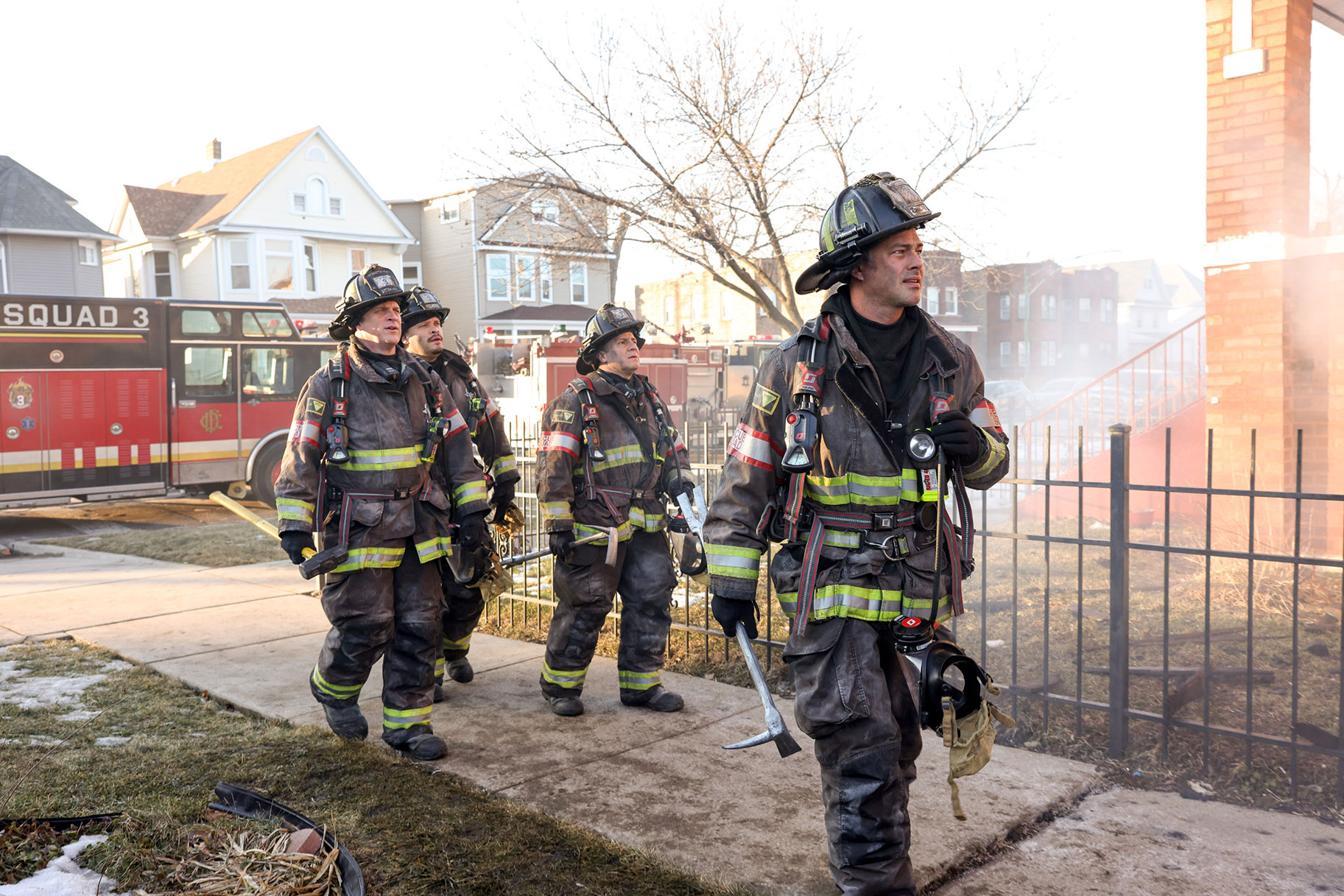The image depicts a tense scene with four firefighters, dressed in full black and yellow gear, looking stern and serious. They appear to be actors from the TV show "Chicago Fire," given the highly detailed and accurate representation. The firefighters are visibly covered in soot and water, likely from a recent fire, and hold tools such as axes, crowbars, and hammers, with respirators draped over their shoulders. They stand on a sidewalk beside a reddish brick building, near a metal fence. In the smoky, overcast background, a fire truck marked "Squad 3" in bold white uppercase letters stands out. Surrounding them is a residential neighborhood where the remnants of a burned house—now just a brick frame and staircase—are visible amidst the haze. A leafless, spindly tree with brown branches further adds to the somber atmosphere.